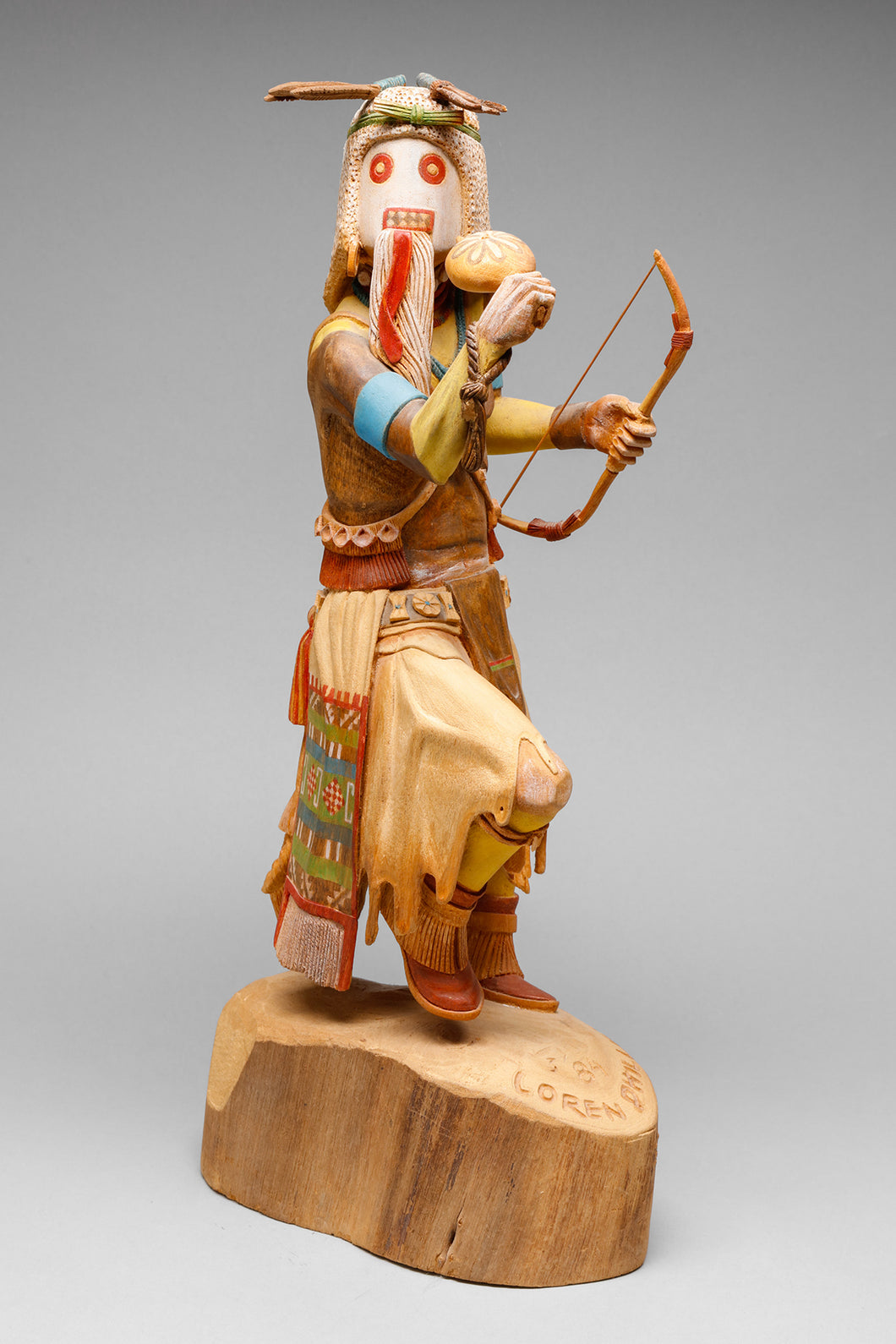This vertically aligned rectangular image showcases a detailed wooden sculpture of a masked figure perched on a round wooden base, which features darker grains on the sides and lighter wood on the top. Partially obscured text on the base reads "Lauren, L-O-R-E-N." The figure represents a warrior or ritualistic character, adorned with a strikingly colorful attire. It has brown boots and brown and tan clothing, with a vibrant scarf draped on its side. The figure's right knee is bent while the left leg remains straight. It is shirtless, with a blue band around its chest. The mask is white with red eyes, gold circles, a rectangular mouth with drawn teeth, and an elaborate helmet-like hat with antler-like brown objects protruding in opposite directions. The figure grips a drumstick with a round top in its right hand and a bow and arrow in its left, and faces towards the viewer while its body is angled to the right. The colors include light blue, orange, tan, beige, brown, and green, set against a gray backdrop. The overall aesthetic evokes a sense of traditional indigenous warrior or ritualistic garb.